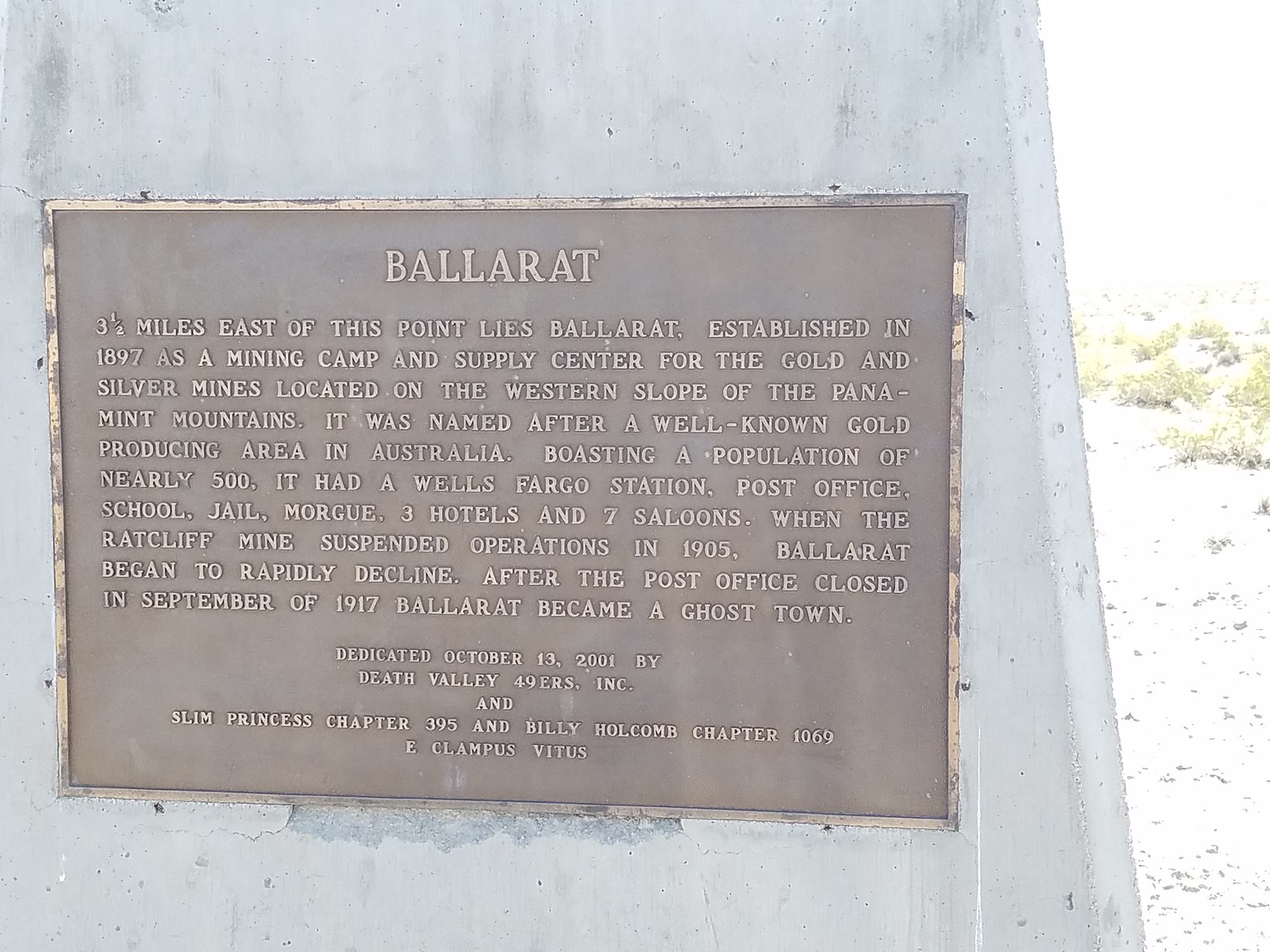This image features a bronze plaque mounted on a grayish marble-like stone base. The plaque is titled "Ballarat" and is dedicated to the now ghost town of Ballarat, located three and a half miles east of the monument's location. Established in 1897 as a mining camp and supply center for gold and silver mines on the western slope of the Panamint Mountains, Ballarat once boasted a population of nearly 500. The town played host to various establishments including a Wells Fargo station, post office, school, jail, morgue, three hotels, and seven saloons. The decline of Ballarat began when the Ratcliffe Mine ceased operations in 1905, and the town ultimately became a ghost town following the closure of its post office in September 1917. The plaque, which is a typical brownish-bronze color, has been dedicated on October 13, 2001, by the Death Valley 49ers, Inc., along with Slim Princess Chapter 395 and Billy Holcomb Chapter 1069, E. Clampus Vitus. The photograph captures this scene on a bright sunny day, evidenced by the overexposed patches of grass visible to the right of the plaque.